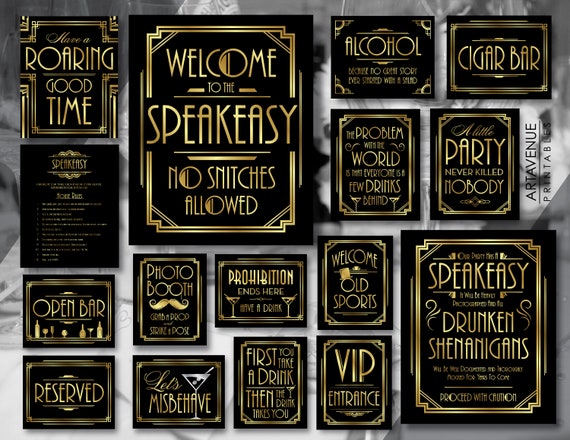This image showcases an array of themed party signs perfectly designed for Great Gatsby or 1920s speakeasy events. Each sign features a distinctive black background adorned with elegant gold lettering and Art Nouveau style borders. Highlighted messages include "Have a Roaring Good Time," "Welcome to the Speakeasy," "No Snitches Allowed," "VIP Entrance," "Let's Misbehave" (accompanied by a martini illustration), and "First you take a drink, then the drink takes you." Additional signs cater to specific party elements such as "Cigar Bar," "Open Bar" (with images of bottles), "Photo Booth," "Reserved," and "A Little Party Never Killed Nobody." The signs are meticulously arranged on a grayish marble background, suggesting an upscale ambiance. This detailed collection vividly captures the opulence and excitement of the Roaring Twenties, bringing a touch of nostalgic charm to any themed celebration.